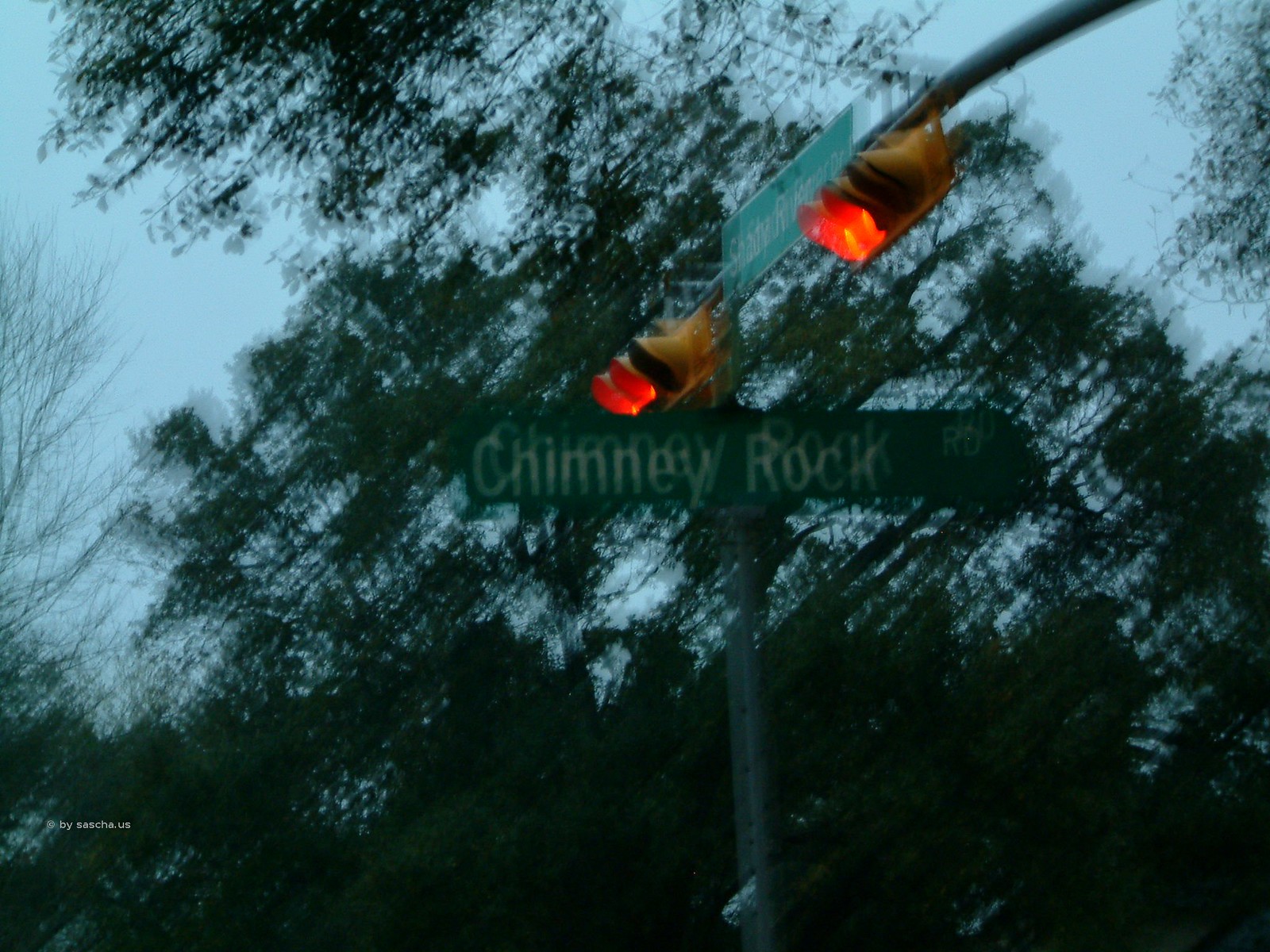In this photograph, taken by SASCHA.US (as indicated by the watermark in the bottom left-hand corner), we observe a street scene marked by unique and intriguing features. Prominently, a silver post in the foreground ascends to support a green street sign with white text, which reads "Chimney Rock Road." Due to significant motion blur in the image, the text on the sign appears doubled, adding a peculiar visual effect.

Another noteworthy element is the traffic light mounted atop the post. Unlike the vertical orientation commonly seen, this traffic light is positioned horizontally, with the red lights on the left. This unusual configuration stands out and may capture the viewer’s interest.

Bright daylight illuminates the scene, with a blue sky providing a serene backdrop. Adding to the natural ambiance, green foliage from nearby trees frames the image. Despite the motion blur, the photograph captures a dynamic intersection, marked by its distinctive street sign and traffic light arrangement.